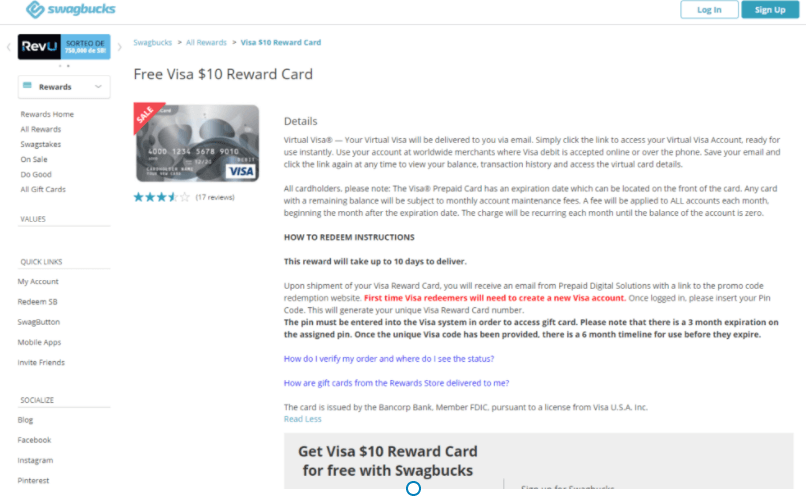This image appears to be a screenshot from the Swagbucks website. In the top left corner, there is a recognizable blue icon accompanied by the blue text 'Swagbucks'. Toward the right, the navigation bar contains two distinct buttons; one with a blue outline and white background that says 'Login', and another with a solid blue background and white text that says 'Sign Up'. A horizontal grey line separates these navigation elements from the main content of the page.

On the left side, there is a sidebar featuring several sections, although they are mostly unreadable. It seems to include a dropdown menu labeled 'Rewards', along with sections titled 'Values', 'Quick Links', and 'Socialize'. On the right, there appears to be a breadcrumb trail, though it is not legible, indicating the navigation path taken to reach this particular page.

The primary focus of the page is a ‘Free Visa $10 Reward Card’ offer. This offer is highlighted with an image of a Visa card. In the top left corner of this image, there is a red triangle marked with white text stating 'Sale'. Below this, the offer boasts a user rating of three and a half out of five stars.

Further down, there are additional informational sections with headings, including one labeled 'Details', although the accompanying text is not readable. There are bolded texts and several links interspersed within the content. At the bottom of the description, a prominent grey box contains bold black text proclaiming 'Get Visa $10 Reward Card for free with Swagbucks'.

Overall, the image captures a detailed promotional offer page on Swagbucks, detailing the availability and specifics of a $10 Visa reward card.